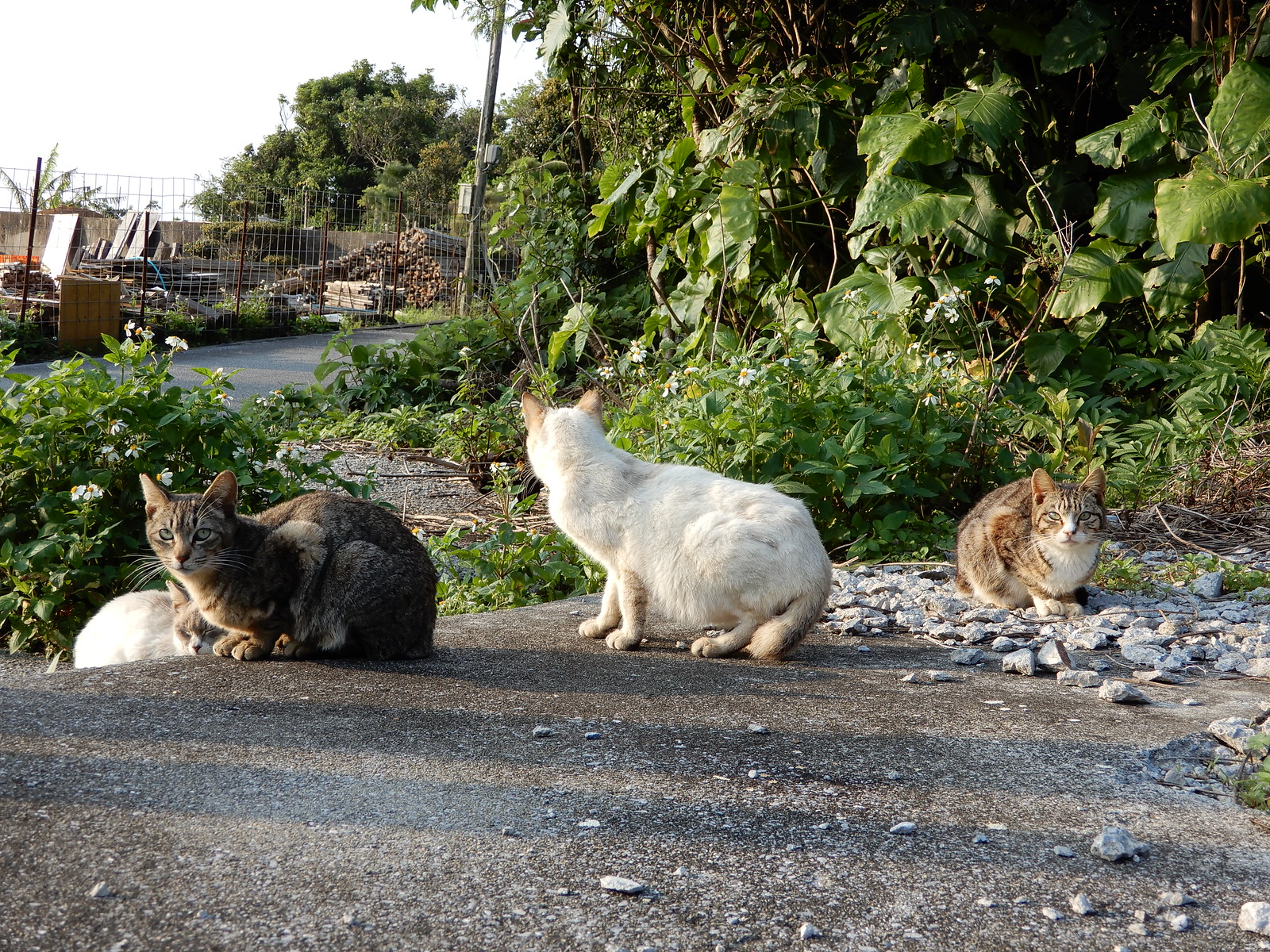In the foreground of the photograph, there are four cats poised on a gray asphalt ground scattered with various white and brown stones. Starting from the left, a cat with a primarily brown body sits among the rocks; it has a white chest, white paws, and green eyes with white fur around its nose. Moving right, a white cat with a brown-tipped tail stands facing away from the camera, obscured partially by the other cats. The next cat, sitting slightly higher on a pile of rocks, is a mix of brown and gray fur with white on its chest and green eyes, directly gazing at the camera. The fourth cat, situated a bit lower, is completely white with a gray head and striking yellow eyes. 

The background of the image features lush, overgrown foliage adorned with white wildflowers that have yellow centers. Dominating the background is a tall chain-link fence, behind which lies what appears to be a lumber yard filled with piles of wood, sheets of metal, and various construction materials. Green trees peek over the high fence, adding more texture to the backdrop. A streetlamp pole with electrical junction boxes is positioned toward the left, near the fence. The entire scene suggests a mix of urban and natural environments, with the cats firmly in focus amid the contrasting settings.